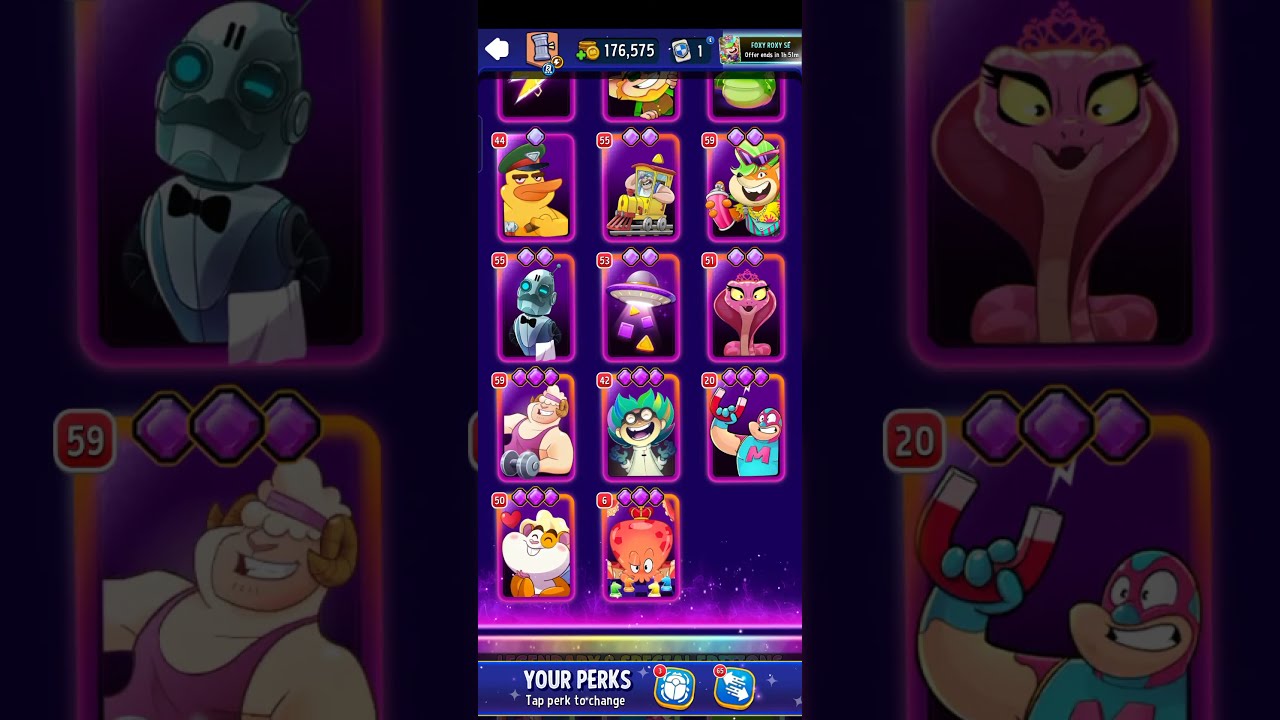The vertical cell phone screenshot captures an image from a mobile video game, centered within a faded, zoomed-in repetition of the same scene for the background. The central game interface showcases a dark blue backdrop with rectangular margins above and below that hold various information. Dominating the center section are rows of square pictures featuring a diverse array of cartoon and video game characters, each framed by a purple border. These characters are arranged in three full horizontal rows and a fourth row containing only two characters, making a total of 14 squares.

Among the characters, notable ones include a thunderbolt, a duck, a snake, a superhero, a spaceship, and a weightlifter. Additionally, specific characters like a robot butler in a tuxedo with diamonds and numerical indicators (55 and 59) and a cobra princess with diamonds and numbers (51 and 10) are prominently visible. The interface is adorned with a variety of vibrant colors like green, yellow, pink, purple, and blue. The top section shows a display of coins totaling 176,575, along with symbols like a lightning bolt, duck in a hat, octopus with a crown, and several other animated figures including a man in a train. The scene vividly represents the colorful and diverse character icons typical of an engaging mobile video game.